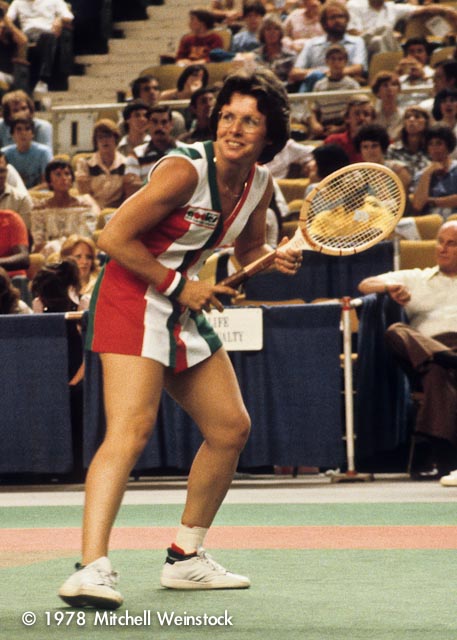In this 1978 photograph by Mitchell Weinstock, tennis legend Billie Jean King is caught in the midst of a match, intently awaiting the next move. Dressed in a striking one-piece tennis uniform adorned with vertical red, white, and blue stripes, she sports white sneakers and glasses, her short brown hair falling just above her shoulders. Billie Jean King is poised with a classic brown tennis racket, her right hand gripping the handle while her left steadies it near the top, her body slightly bent forward in anticipation. The tennis court, possibly artificial grass, forms the stage where she stands with legs apart, ready for action. Behind her, a vigilant crowd fills the arena, their eyes glued to the unfolding game. To her right, an official in a white shirt and brown pants sits outside the match area, checking his watch. The photo also features the text "© 1978 Mitchell Weinstock" in the bottom left corner, preserving this historic sporting moment.